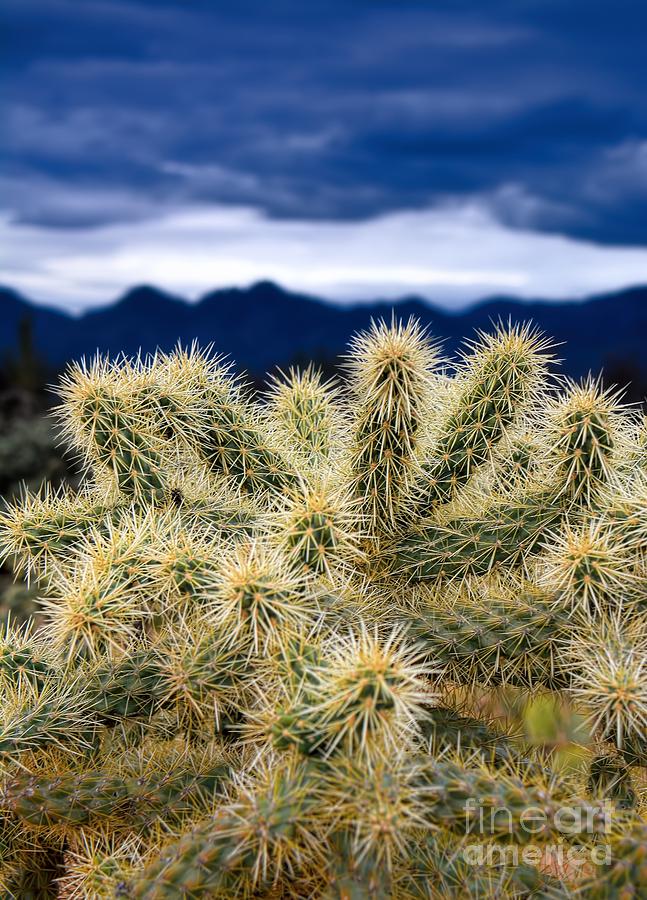This vertical-rectangular photograph captures a close-up of a cactus with a blurred mountainous background, likely set in a desert region such as Arizona. The cactus dominates the frame with its light green, bush-like structure comprised of numerous long, round branches, some of which are curved. Each branch is densely covered with inch-long, yellowish needles that fan outwards. The background features a dark blue mountain ridge, which is blurred to emphasize the foreground cactus. Above the mountains, a gradient sky transitions from a light blue near the horizon to medium-tone clouds, with darker clouds higher up. In the lower right corner, the words "Fine Art America" appear in white or grayish-transparent lettering, suggesting this is a photograph from a fine art collection.